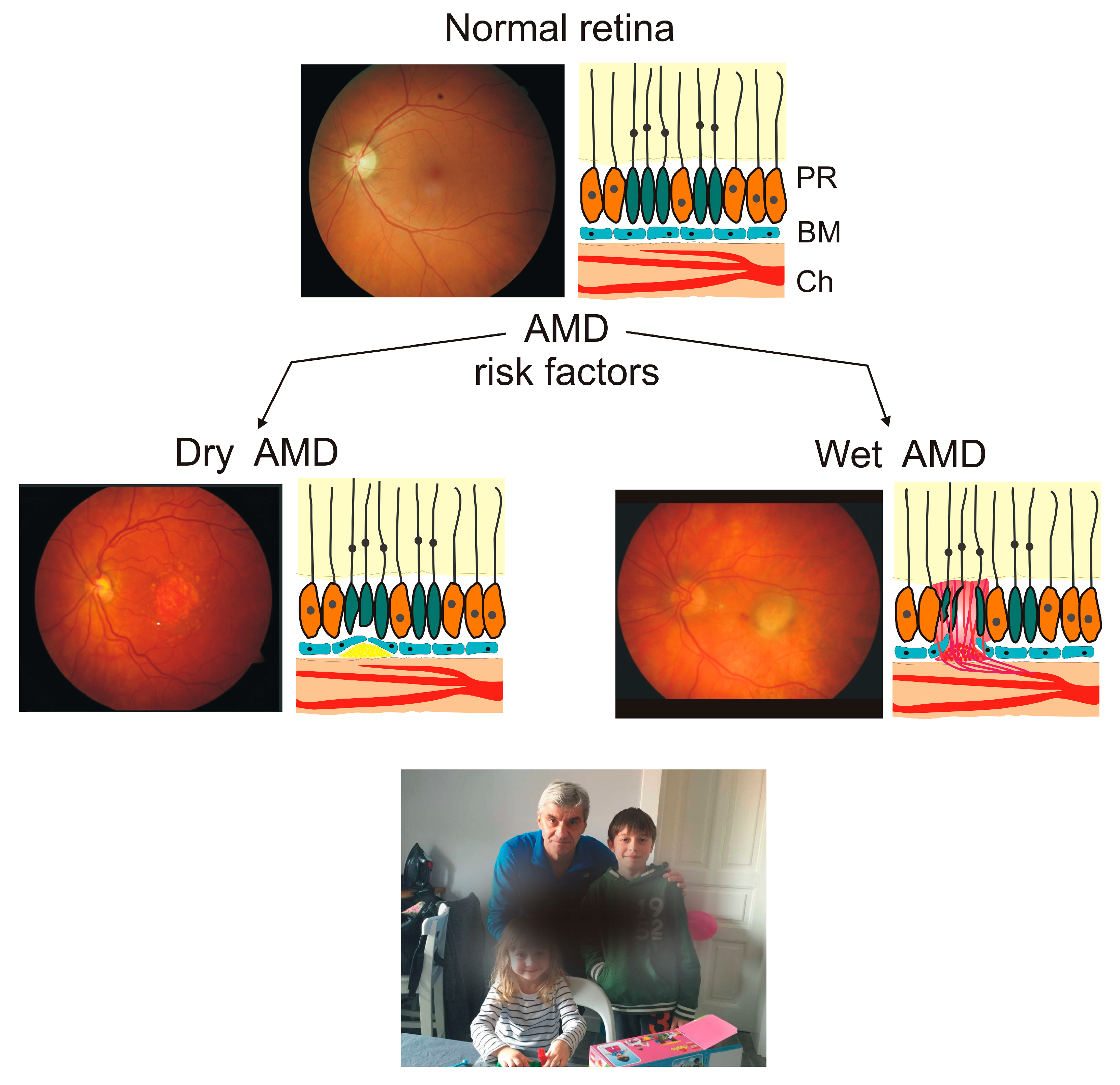The multi-paneled image provides a detailed comparison and illustration of retinal health and disease progression. At the top, the chart contrasts a normal retina with depictions of diseases like dry Age-related Macular Degeneration (AMD) and wet AMD. The left panel features an actual image of a healthy retina, showcasing its vibrant orange hues interspersed with white and red veins, and a darker central region. Next to this is a schematic drawing of the retina's cellular makeup, labeled with PR (photoreceptors), BM (Bruch's membrane), and CH (choroid).

Beneath these, the chart delineates the changes in the retina due to dry AMD and wet AMD. For dry AMD, another retinal image is provided alongside an illustrative degradation of the retinal cells. For wet AMD, similar depictions highlight the disease's progression, marked by notable bleeding and damage in the retinal tissues.

At the bottom of the image, a photograph of a man and two children is partially obscured by a dark gray spot, simulating the central vision loss experienced by individuals with AMD. The man, wearing a blue shirt, stands beside a boy in a green hooded sweatshirt and a girl in a white shirt with dark stripes. This visual distortion emphasizes the impact of AMD on daily life and clear vision.